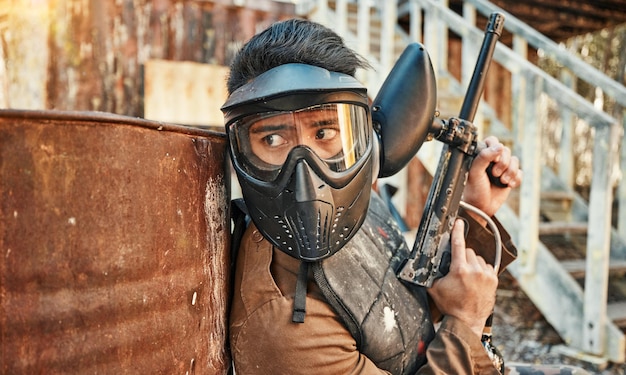In the image, a paintballer with visible black hair and a fully covering mask—featuring transparent goggles over the eyes and breathing slits below—kneels behind a rusted barrel. The paintballer dons a vest with noticeable paint splatters over a brown jacket, possibly made from cloth or leather, and stiff chest armor for added protection. The paintballer holds a paintball gun with a prominent hopper attached to the top, aimed at a slight upward angle, and appears to be gazing seriously or worriedly off to the side. The background reveals a rundown shed or house with grubby white stairs ascending behind the subject.